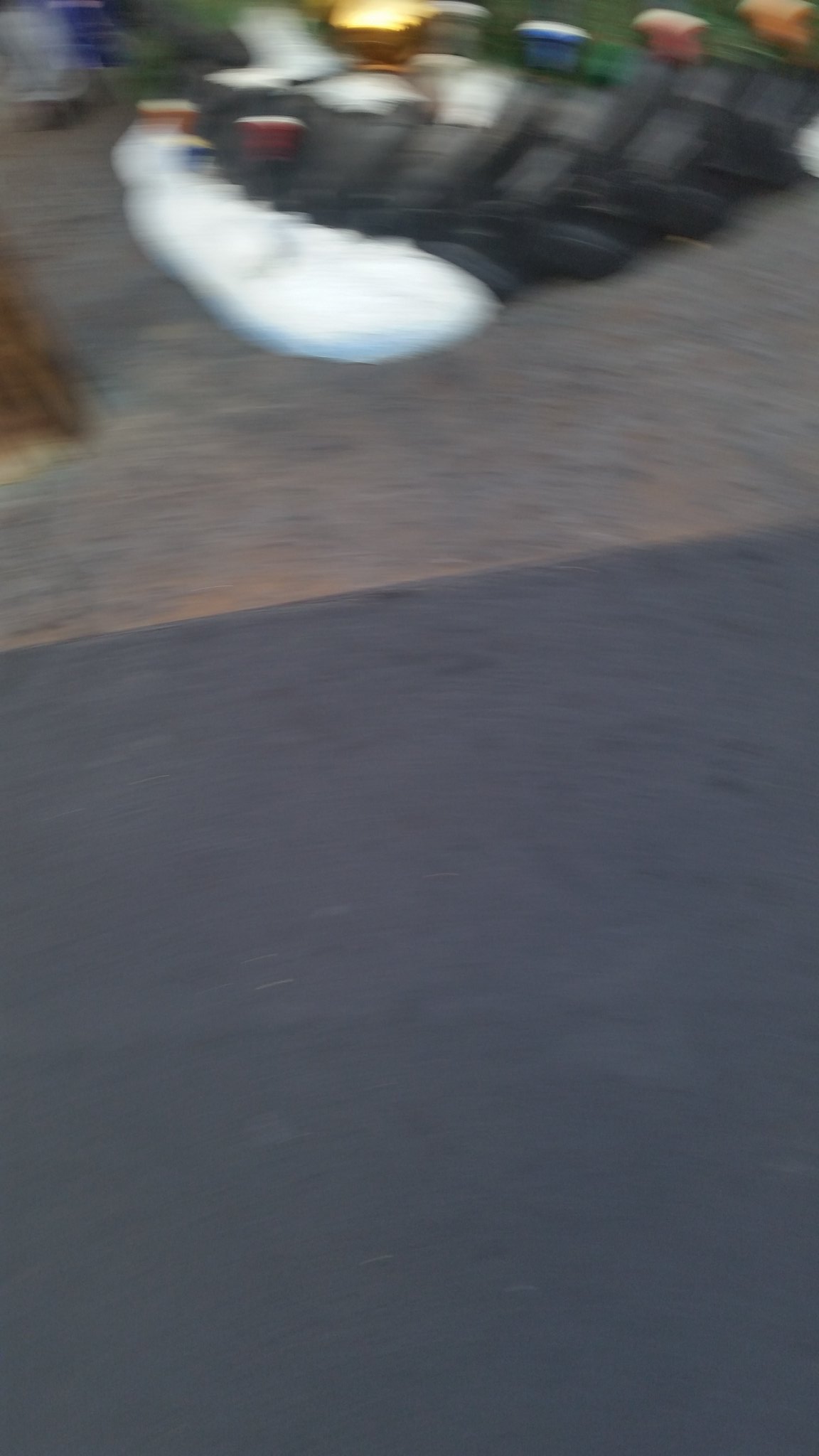The photograph is a very blurry color image with a vertical orientation. The lower half of the image is predominantly black, providing a stark contrast to the upper section, which transitions into a brown hue. At the very top edge, there is an indistinct object that features a base which appears to be white, possibly resembling snow. This object is primarily a dark brownish-green and is adorned with multicolored circular decorations in red, blue, and gold. The image lacks any visible people, animals, buildings, signs, or writing, maintaining a focus on this enigmatic, festively adorned object in a seemingly natural or outdoor setting.